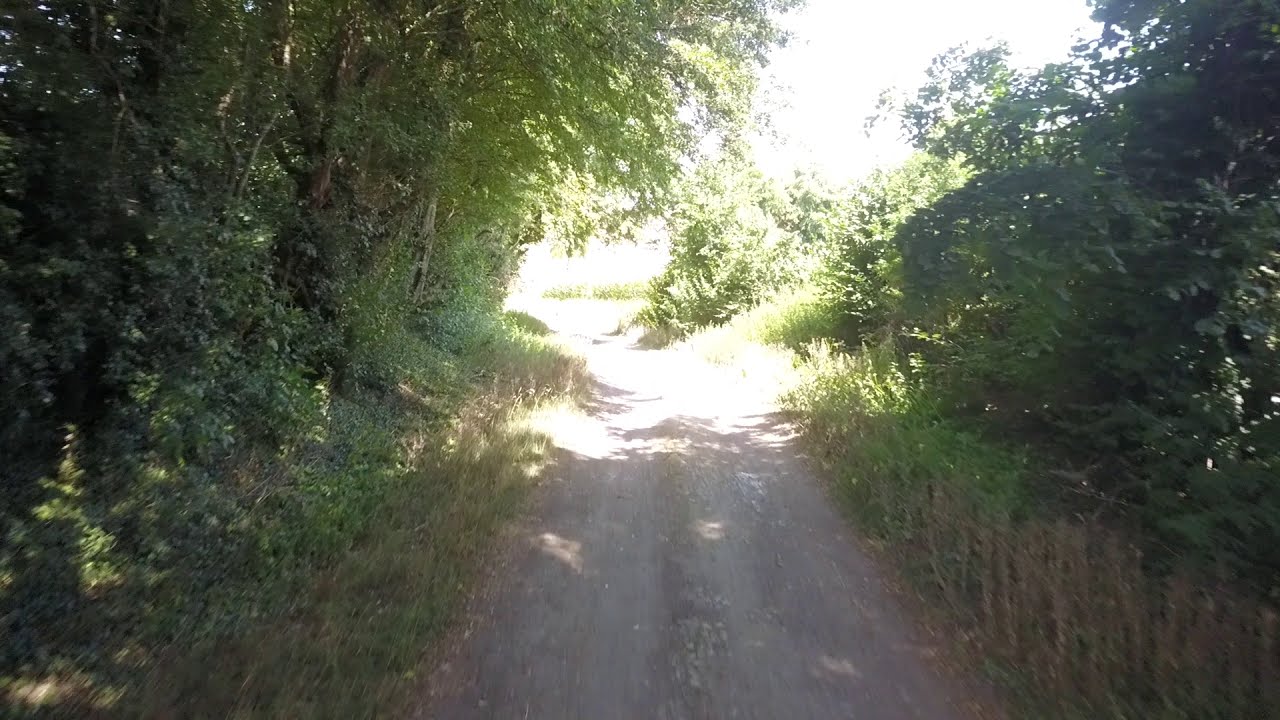The image captures a scenic country path, likely a dirt road or driveway, stretching straight ahead from the bottom of the photograph. The pathway exhibits signs of human activity and is narrow, appearing fit for only a single vehicle. On the left side, densely packed tall green trees and grass border the road, while the right side features patches of tall brown grass with green trees visible beyond them. Heading towards the back of the image, the path is brightly illuminated by sunlight, causing a lack of detail and a blown-out effect towards the horizon. The bright white sky further accentuates the brightness of the day. Some lighter-colored leaves in the greenery suggest the photo might have been taken in late summer. The road shows a distinct bump or discoloration running down the middle, giving an impression of a split. Overhead, the camera is shaded by the surrounding trees, adding to the contrast with the sunny backdrop.